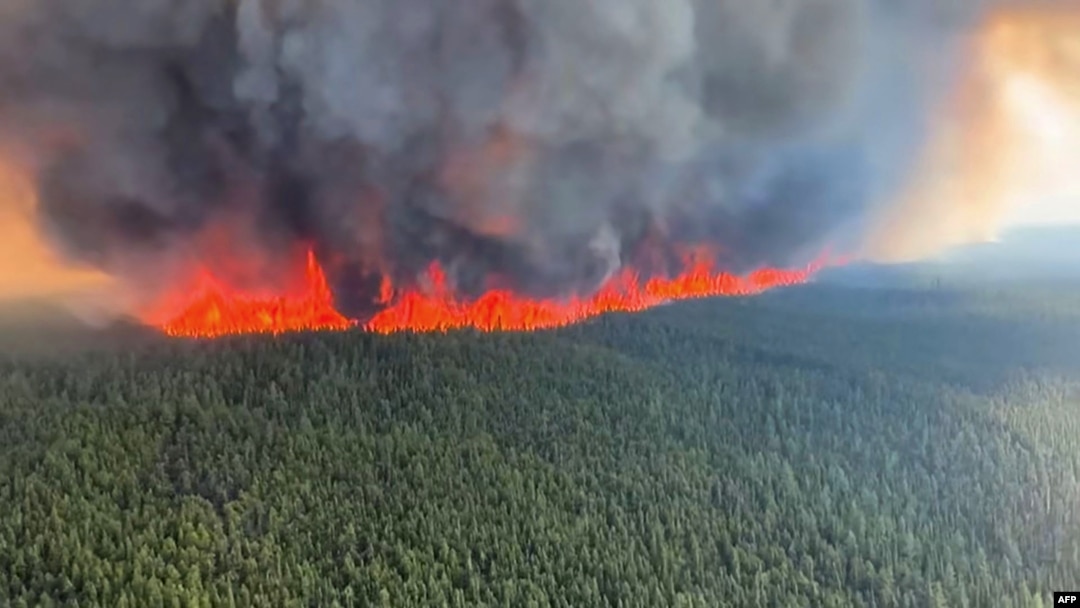The image, taken from an aerial perspective, depicts a very dense forest engulfed in a massive fire. The forest, uniformly green and seemingly endless, is made up entirely of trees with no visible signs of human habitation. Bright red and orange flames emerge at the top of the forest, creating a striking contrast against the green canopy. The fire appears to stretch across the landscape, encircling the forest in a continuous line of intense heat. Above the flames, thick billows of gray, black, and white smoke obscure the sky, indicating the severity of the blaze. In the bottom right corner, the image is marked with the label "AFP" in small white letters, suggesting an official source. Overall, the image captures the dramatic and destructive impact of the wildfire as it consumes the forest and spreads smoke throughout the area.